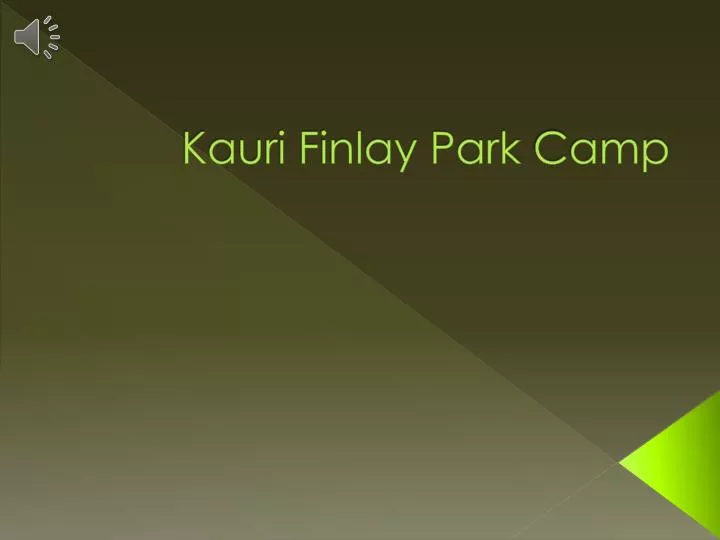The image displays a computer screen featuring a PowerPoint slide with a predominantly green color scheme. In the upper left-hand corner, there is a gray speaker icon, indicating audio functionality. The slide is divided into gradients of green, with a darker olive triangle occupying the upper and right sections, and a lighter olive triangle in the bottom left. Near the bottom right corner is a small, bright fluorescent green triangle embedded within the larger dark olive triangle. About a quarter of the way down from the top, text in light green reads "Kauri Finlay Park Camp," with the first letters capitalized (K, F, P, C) and written in a larger font size, approximately 20-point. The overall design employs a geometric pattern with varying green shades, creating a visually cohesive look.